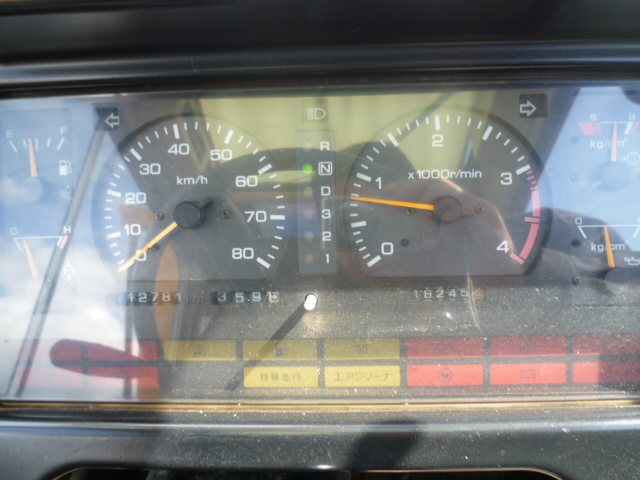The image captures a close-up view of a car dashboard. Dominating the scene are two prominent circular dials: the left one displaying the car's mileage and the right one indicating the engine's RPM. Reflected in the dashboard's glass is the photographer's hand, suggesting the photo was taken in close proximity. Centrally, a gear indicator shows the car's current state—whether it's in reverse, neutral, drive, or one of the lower gears (third, second, or first). Below this, a digital readout reveals the car has over 102,000 miles on it. Arrayed along the bottom of the dashboard are various warning lights and sensory indicators in red and yellow. Although the labels on the buttons are not entirely clear due to the language barrier—they appear to be in an Asian script—some symbols can be vaguely discerned, such as a potential battery light, although their exact functions remain ambiguous.